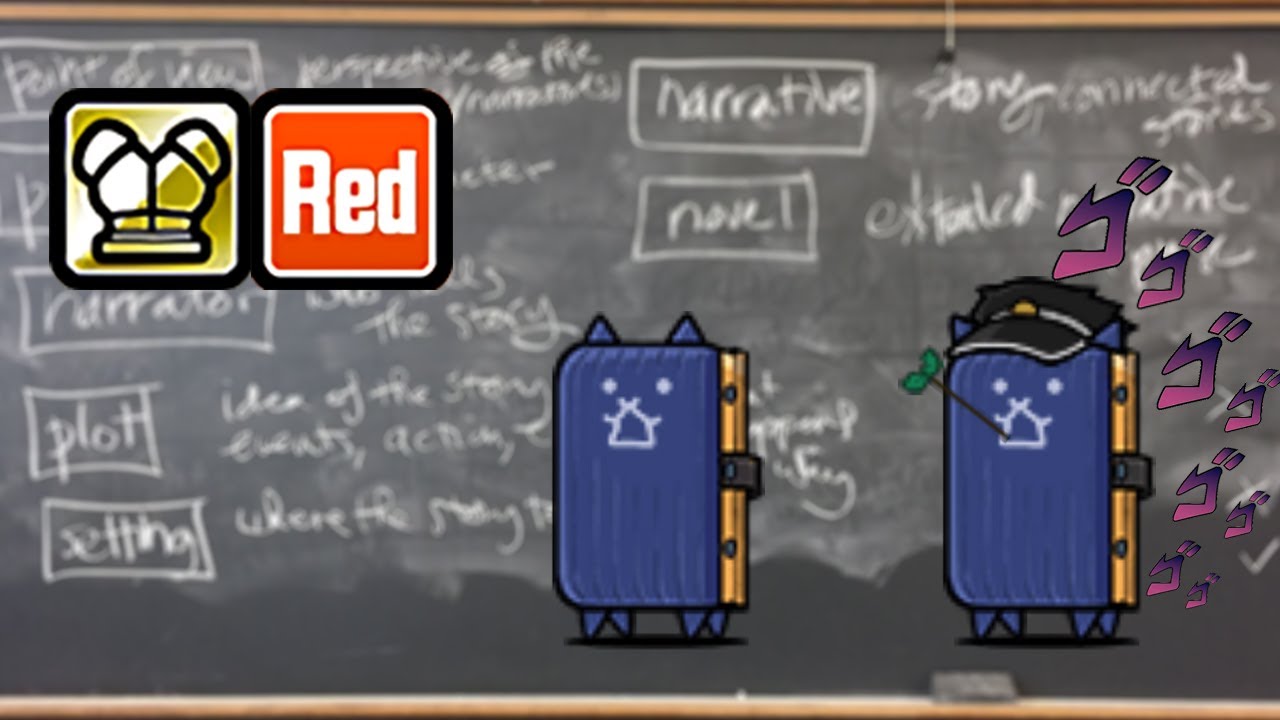This cartoon-style image features a slightly blurry blackboard as its background, filled with white chalk writing that includes terms like "narrative," "plot," "setting," and "novel." Located in the top left corner of the blackboard are two prominent logos: a golden emblem with a chess piece design on the left, and a red box with the word "red" written in white letters on the right. In the foreground, two blue suitcases designed to resemble cats are showcased. The suitcase in the center has a simple cat-like face with blue ears and a yellow outline. The suitcase to its right sports a black police cap, a twig with leaves in its mouth, and features similar cat-like facial details. To the right of these suitcases are a series of purple Japanese characters that read "go go go go go go go go," presented in a dark to light purple gradient. The entire scene is contained within a horizontal rectangular frame, blending cartoon and possibly digital elements seamlessly.